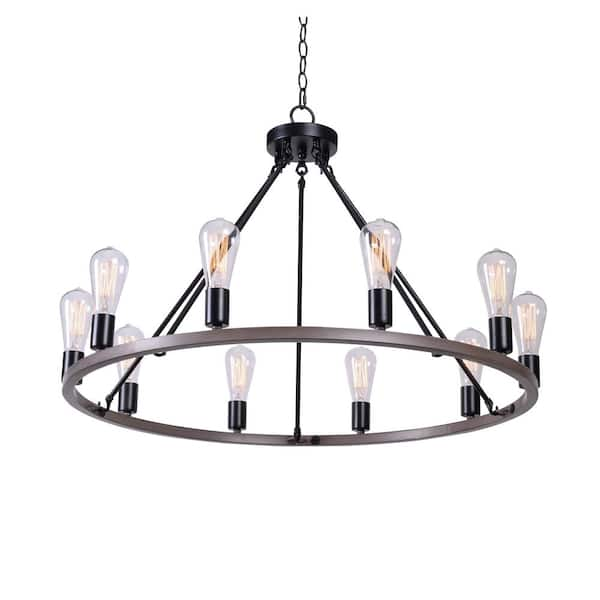This photograph showcases a rustic, country-style chandelier suspended by a chain composed of six links. The chandelier is predominantly black and is designed with an industrial aesthetic, characterized by 10 light bulbs each resembling vintage tungsten bulbs with visible yellowish-gold filaments inside. These light bulbs are evenly spaced around a circular ring, lending an orderly and symmetrical appearance. The ring itself is held aloft by a combination of five black beams, extending from the circular light fixture up to a central cylindrical piece, which ensures structural support. The entire fixture is attached to the ceiling via a chain connected to a circular platter. The background in the image is completely white, highlighting the contrast between the black structural elements and the softly glowing light bulbs.